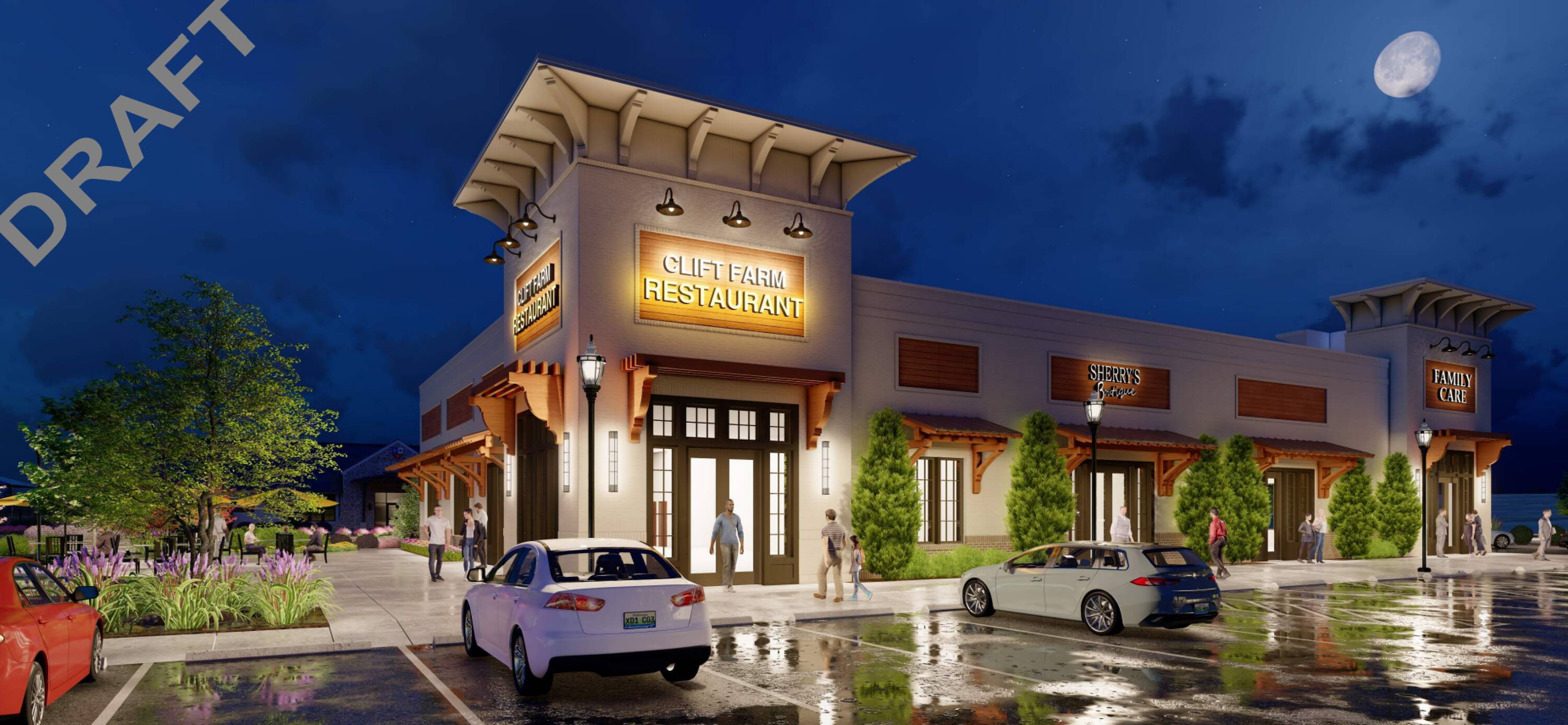The image showcases a photorealistic representation of a twilight scene featuring a mini mall with a prominent restaurant called Clift Farm Restaurant at the corner. The sky above is a deep blue, characteristic of dusk, with dark blue clouds and the moon visible in the upper right corner. A watermark with the word "DRAFT" in uppercase gray letters stretches diagonally across the upper left. The mall also houses Sherry's Boutique and Family Care, with all signs illuminated. The entrance to Clift Farm Restaurant is notable, with double doors framed by black trim and lights illuminating the sign above. The parking lot in front is slick with rain, reflecting lights from the buildings. Three cars—a modern white station wagon, another white car a few spaces down, and a red car—are parked in the lot. People are seen walking on the gray sidewalks, which are lined with green plants and purple flowers, and multiple trees contribute to the scene’s vivid detail.